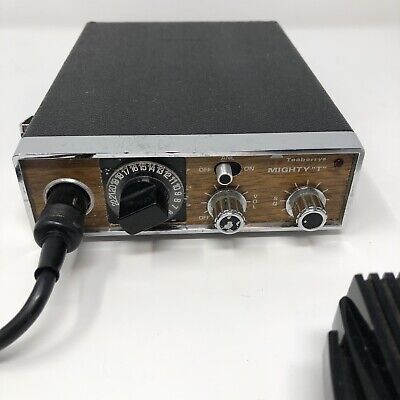The image depicts an older-style CB (citizen's band) radio, recognizable from its rectangular, black body resting on a white table. This vintage device features a distinctive front panel with a combination of black, silver, and walnut brown accents. The controls are neatly arranged, with five knobs dominating the front. Starting from the left, a black cord is attached, likely for power or an external connection. Adjacent to this is a numbered dial, with the highest visible number being 22, indicating it’s likely used for frequency or channel selection. The middle knob controls the power, marked with "ON" and "OFF" positions. The volume is adjusted by the next knob, labeled "VOL" with an associated "OFF" marking. To the far right, there are additional knobs, one of which bears the label "MIGHTY" with a "T" in quotations above it, although its specific function is unclear. There is also an “on/off” switch, and switches for functions like squelch. The front panel is trimmed in silver metal along the edges, while the area around the dials features a walnut brown trim, giving it a classic, retro appearance. The background includes a light gray surface with a lot of white light, making the radio stand out prominently.